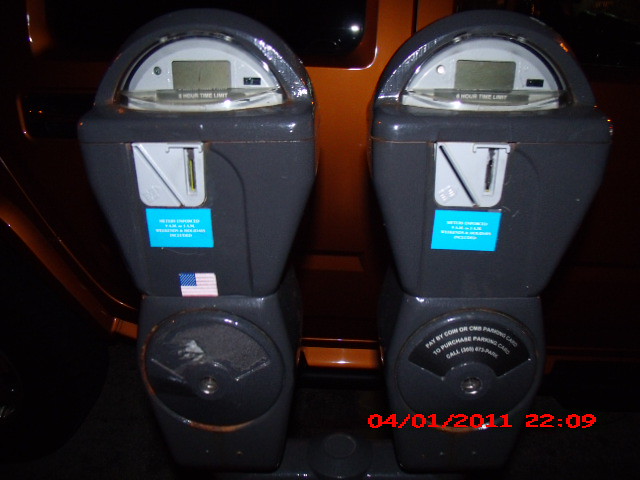In this night shot dated April 1st, 2011, at 22:09, two gray metal parking meters stand next to an orange vehicle, possibly a Jeep. The meters are positioned very close together and are adorned with various stickers. Notably, the meter on the left features an American flag sticker, while both meters have blue stickers beneath their coin slots. The coin slots, designed to collect payments, do not display any operational graphics. The meters exhibit a shiny gray paint and a circular top that should house a needle, although none is visible. The meters' exteriors include silver metal components seen through clear sections. The background is dark, and the image is slightly out of focus, highlighting the reflective surfaces of the orange vehicle next to them.